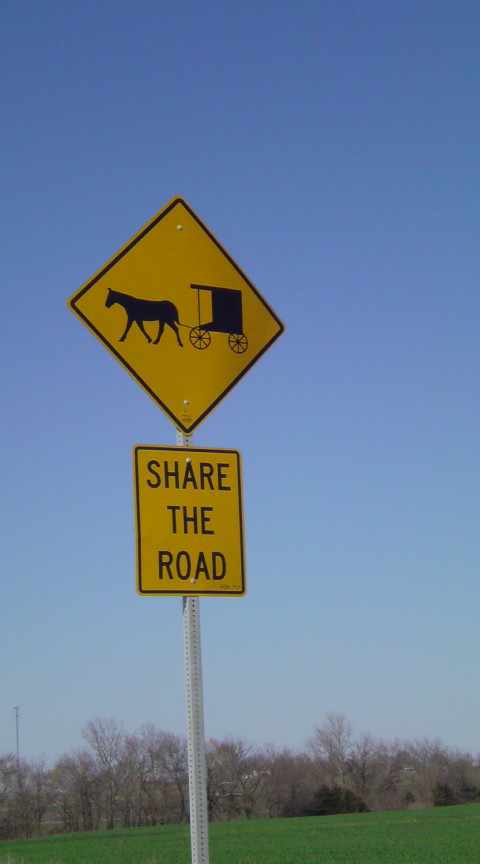This photograph, captured in a vertical orientation, showcases a road sign against an outdoor backdrop. The background displays a vibrant blue sky, accentuated by a row of mature trees, bare of leaves, standing tall. A lush green field stretches out beneath them. From the ground rises a squared metal post, to which two signs are affixed. The top sign, diamond-shaped and safety yellow, features the silhouettes of a horse and buggy. Beneath it, a rectangular sign with black text reads "Share the Road." This image effectively conveys an important traffic advisory in a scenic rural setting.